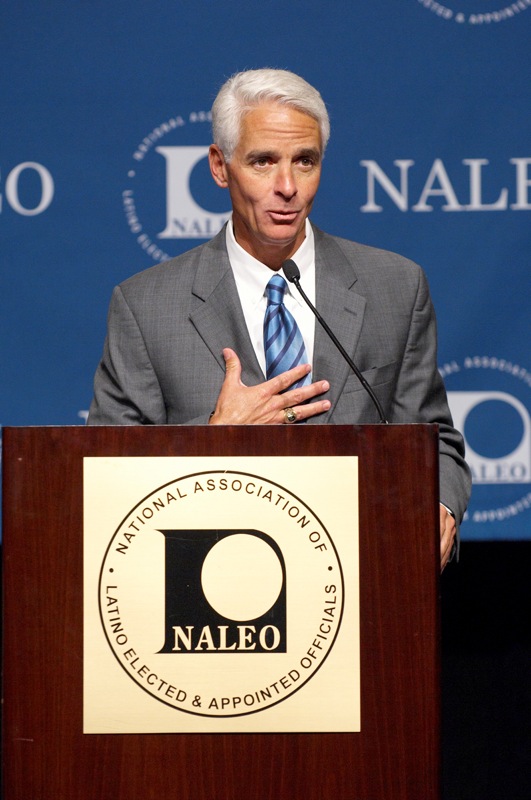The photograph captures a man with short gray hair and a thin face, seemingly in his late 40s or early 50s, standing behind a substantial brown podium that spans from the left edge to the right edge of the image and extends off the bottom of the frame. The podium features a light-colored sign prominently displayed on the front. This sign has a distinct circular emblem; inside the circle, against a black background, the acronym "N-A-L-E-O" is written, while the perimeter of the circle reads "National Association of Latino Elected and Appointed Officials". The man is wearing a gray suit, a light-colored shirt, and a light blue striped tie with dark blue stripes. He stands facing forward with a slight rightward angle. His right hand is positioned in front of his chest, revealing a ring on his ring finger, while his left arm rests down at his side. A microphone stands before him on the podium. The background is a blue wall adorned with repeating "N-A-L-E-O" symbols and the same circular design that appears on the podium's sign.